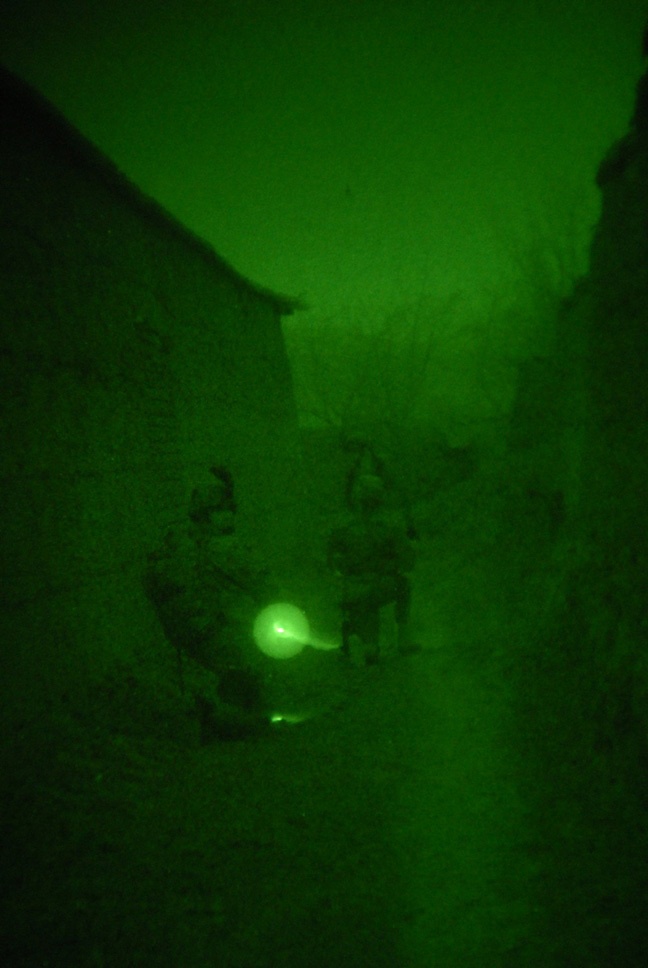This infrared military scene, cast in a vivid green night-vision hue, captures three soldiers in a tactical formation. The central figure, standing at the forefront with a large backpack, turns slightly backwards, his face partially illuminated by the flashlight held by the soldier behind him. This intense beam obscures some details, creating a stark contrast against the night-vision backdrop, which fades into darker shades of green toward the top. The two soldiers in the rear are kneeling, one also orienting backwards. They are all clad in full camouflage gear, complete with helmets and backpacks.

The terrain is a mix of dirt and scattered vegetation, framed by the impression of barricades on either side which might be small walls or buildings, shifting into obscured shapes under the greenish glow. Slightly faded trees loom in the background, and a path appears to cut through the center of the scene, adding depth by leading the viewer's eye further into the composition. The perspective suggests the photo could have been snapped from a vantage point within a first-person shooter game, contributing to its dark, immersive quality.